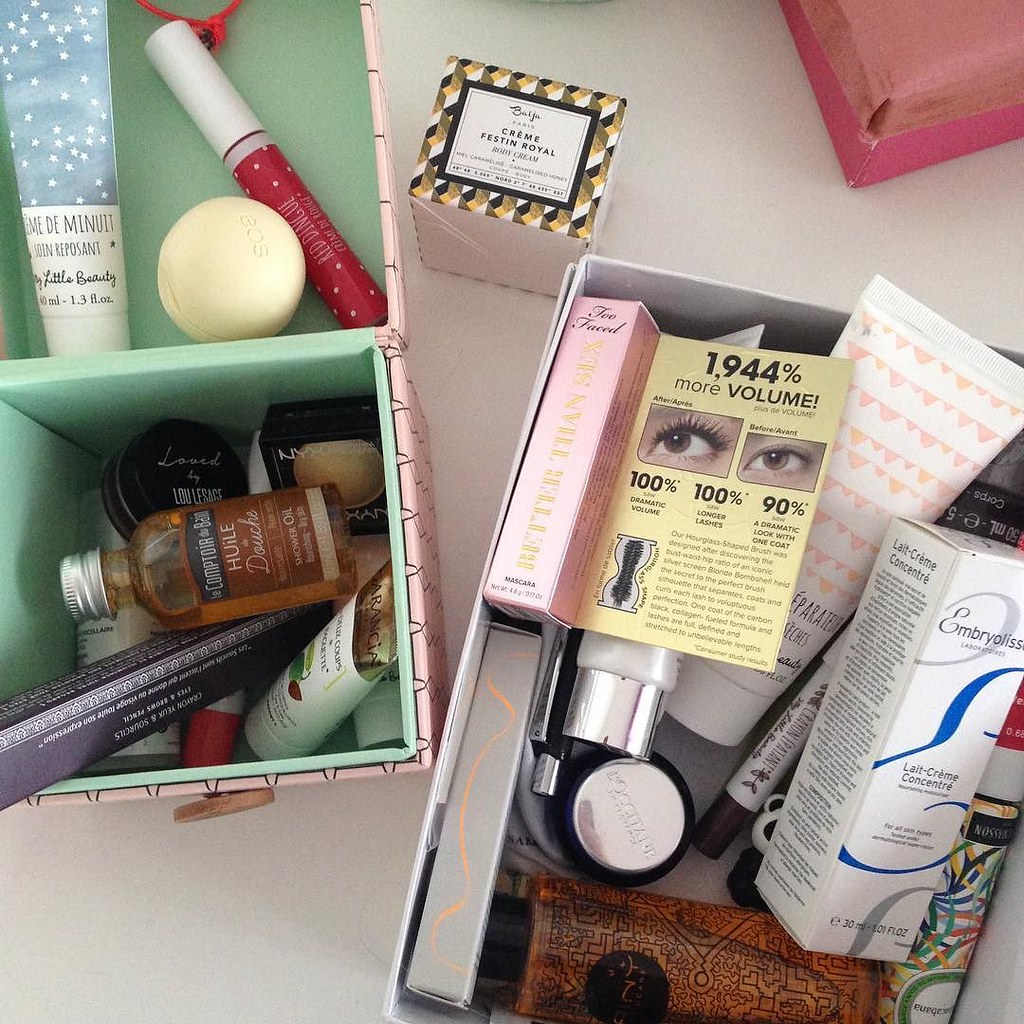The image showcases a top-down view of several box containers filled with skincare and makeup products, meticulously arranged on a gray table. 

On the right side, there is a box with gray outer edges containing various items. Among them, a white rectangular package stands out alongside several makeup containers. Below, there's a distinctive brown bottle adorned with black designs and capped with black. Adjacent to it are a gray container on the left and a pink one in the front. A notable yellow sign marked "1944% more volume" with illustrations of eyes adds a pop of color to this arrangement.

To the left, a mint green square box neatly holds six skincare products. In front of this box, another mint green container is visible, housing three additional products and a noticeable bright red string emerging from the top. 

Finally, one more box to the right features a white label with a yellow, white, and brown checkered design. Atop this box is a pink object with varying shades of pink. The entire assortment is neatly placed on a gray tabletop, providing a subtle yet elegant background for the vibrant display of beauty products.